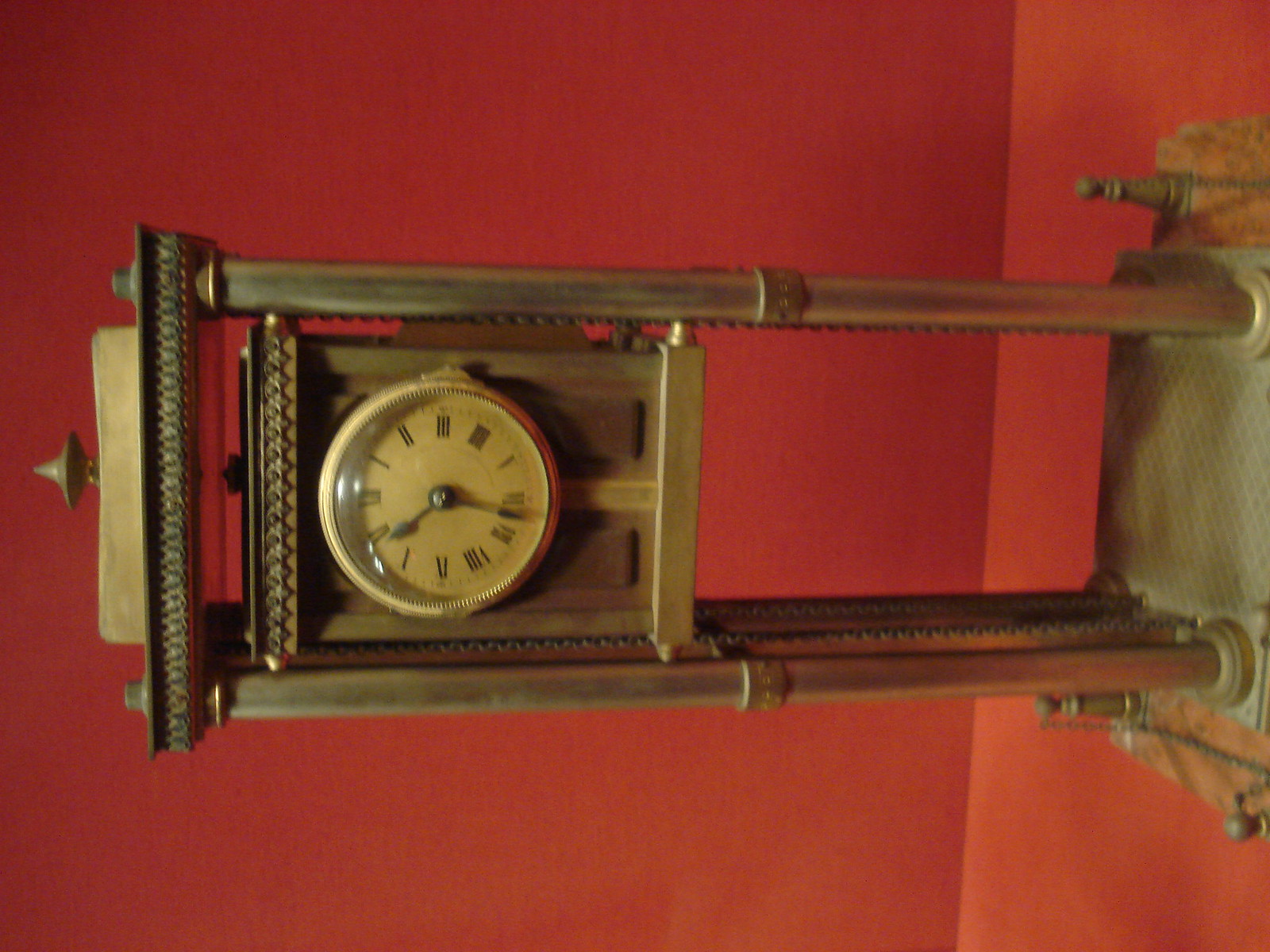This image showcases a vintage-style brass clock with a lavishly ornate design. The clock boasts a rich, brassy golden hue and is mounted on a cubic base supported by four slender legs. Atop the clock is an intricate, pointed lid adding to its opulent charm. The clock face, circular in design, features a golden background with a gold rim. The time is marked by black Roman numerals, complemented by elegant black hour and minute hands. The clock stands against a striking red backdrop. The photograph is displayed in landscape mode, although it was originally shot in portrait orientation, resulting in a 90-degree tilt to the left.